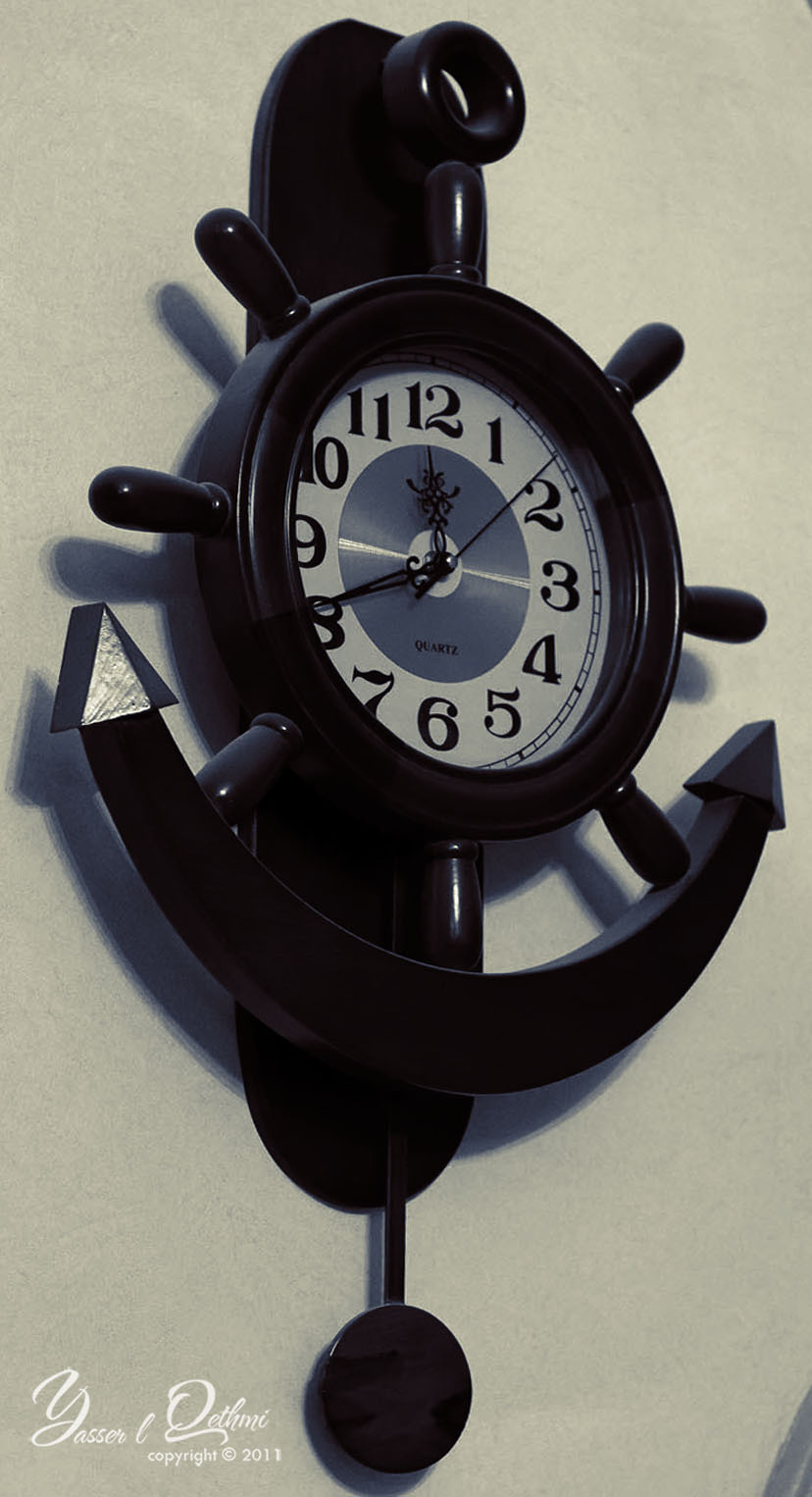This image features a black clock with numerals 1 through 12 and black hands. Positioned just below the clock is a sign resembling an upward-curved smiley face, also in black. At the bottom of the clock, there's a mechanism that appears to chime on the hour. The clock and its elements evoke a maritime theme with a black ship's wheel design, complete with handles that mimic a helm. This maritime clock is mounted on a stark white wall. In the bottom corner of the image, a copyright notice reads "Yassi Othein, 2011," indicating the photographer's name and the year the image was taken.